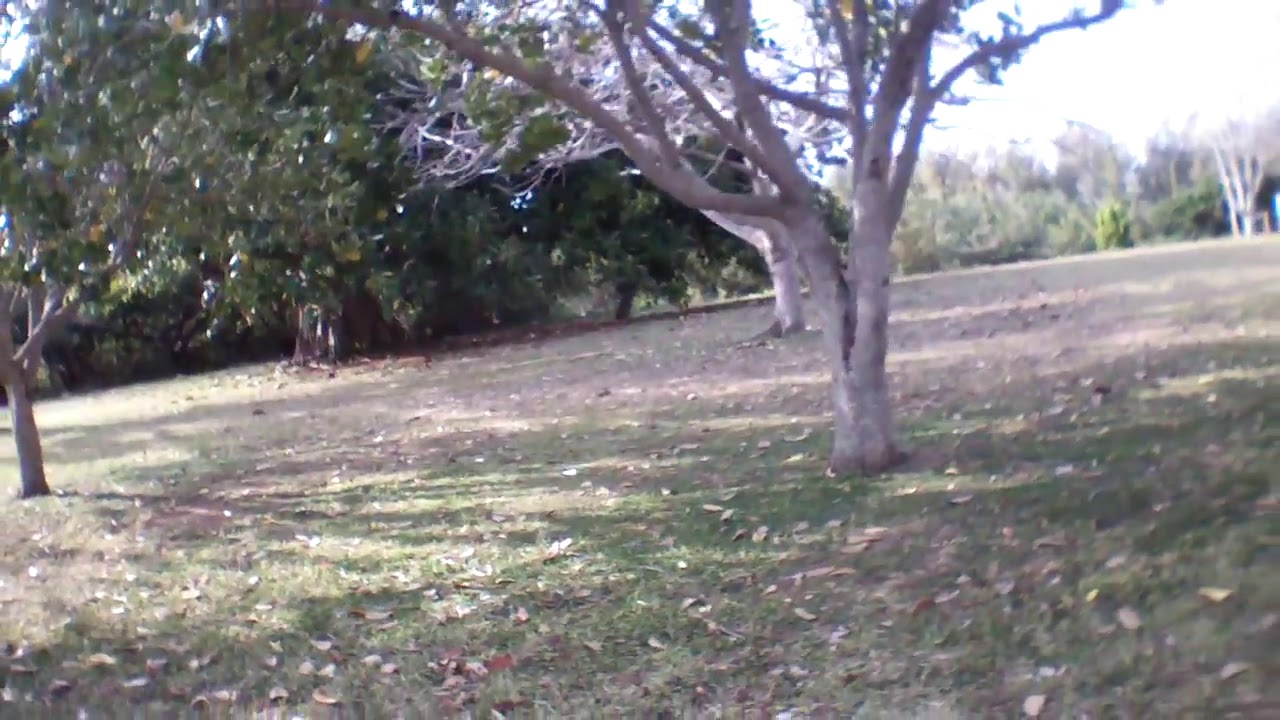This horizontally rectangular, full-color photograph, taken outdoors on a sunny fall day, captures a somewhat faded and slightly out-of-focus scene of a park. The foreground features a neatly mowed lawn with green and brown patches, indicating areas of healthier and dehydrated grass respectively, interspersed with numerous dead leaves. Dominating the scene is a light brown tree near the center with extensive branches and green leaves. To the left, two almost leafless trees stand out, while the background shows a dense cluster of lush green and colorful fall foliage. Sunlight streams through, creating patches of light on the ground. Additional trees are visible to the left and right. In the upper left corner, a bicycle is parked under a tree, and in the upper right corner, there is a small white structure resembling a tower on a white base. The photograph depicts an undisturbed, tranquil park setting in nature with no visible people or animals, capturing the essence of the wilderness.